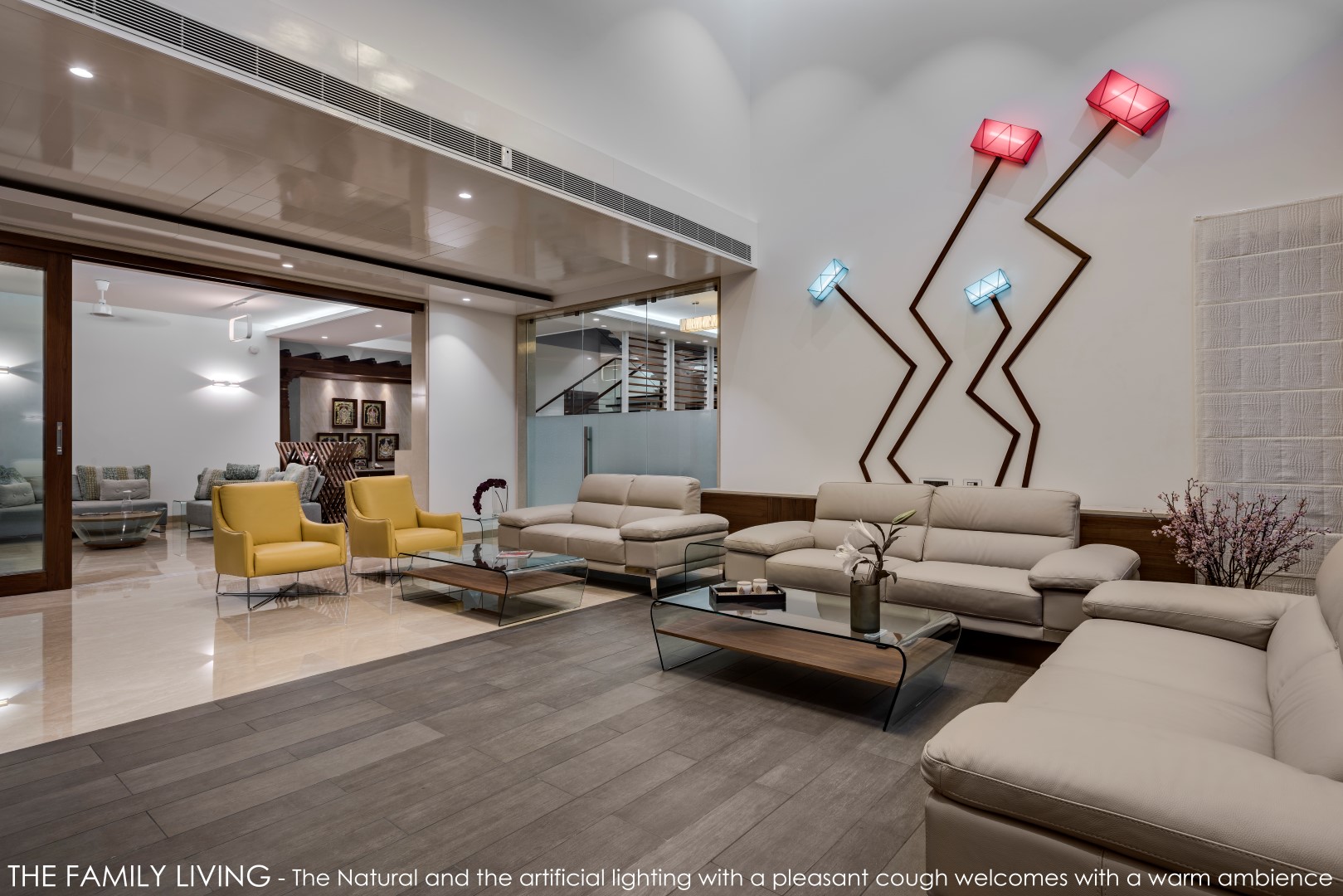This image captures a spacious, contemporary living room with a sophisticated ambiance, potentially an upscale home or a modern office lobby. Dominated by neutral tones, the room features tan-colored walls, and the majority of the seating includes beige sofas and loveseats, complemented by two mustard-yellow chairs. Central to the seating area are two medium-brown wooden coffee tables with glass tops.

The flooring transitions from a darker, horizontal plank wood in the main room to a glossy, tile finish leading to an adjacent space. The back wall is adorned with striking abstract art: jagged zigzag lines in brown and black, culminating in illuminated boxes—two small blue boxes and larger reddish-pink ones, enhanced by LED lights. Additional features include a massive pocket door, a glass partition separating multiple rooms, and numerous wall-mounted pictures, indicating a seamless blend of privacy and openness.

The rooms are well-lit naturally and artificially, casting soft shadows and reflections, enhancing the inviting yet modern atmosphere. A caption at the bottom reads, "The family living, the natural and artificial lighting with a pleasant cough, welcomes with a warm ambience," further emphasizing the room's harmonious blend of comfort and contemporary design.